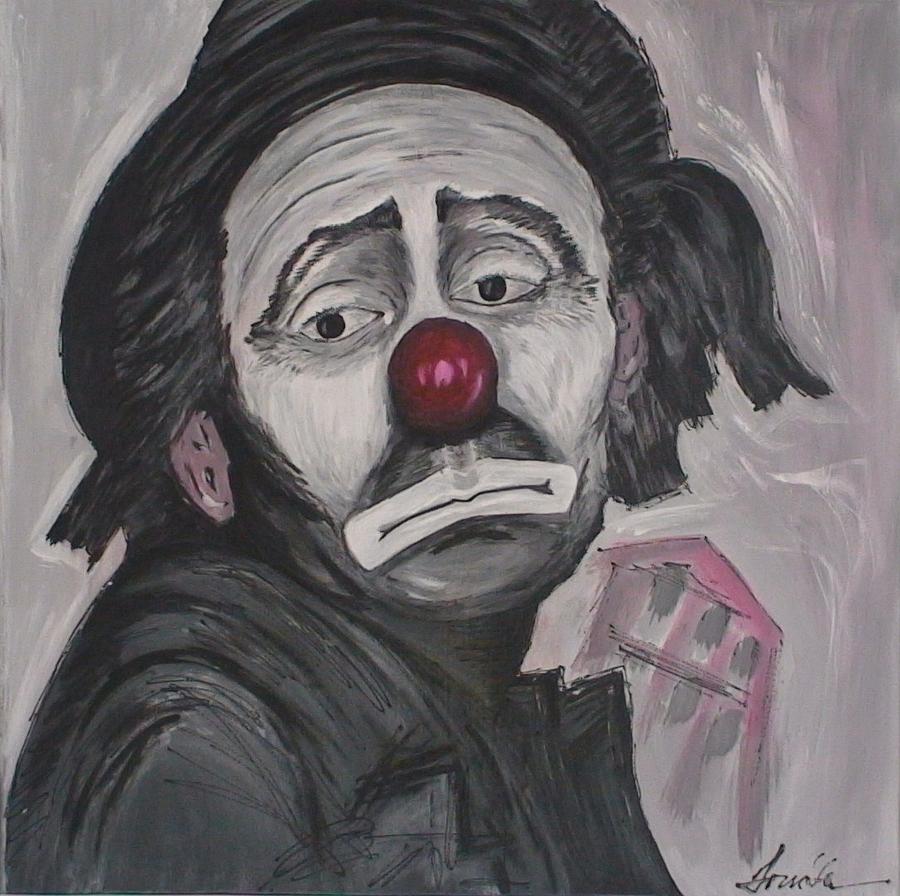This detailed artwork is a charcoal drawing of a sad clown, predominantly in monochrome shades with selective use of color. The clown's expressive face is painted white with emphasized white lips and a prominent red nose, which resembles a shiny cherry. His somber expression is highlighted by his downturned mouth and eyes that look off to the left, while his head faces forward. The clown is adorned with a black hat on top of black hair and wears a black jacket with visible lapels. The composition shows a minimalistic house situated in the bottom right corner, rendered in muted tones of pink, grey, and white. In the same corner sits an indistinct, squiggly signature, potentially reading "Forsoffer." The background of the piece is predominantly grey, accentuating the melancholic mood of the drawing.